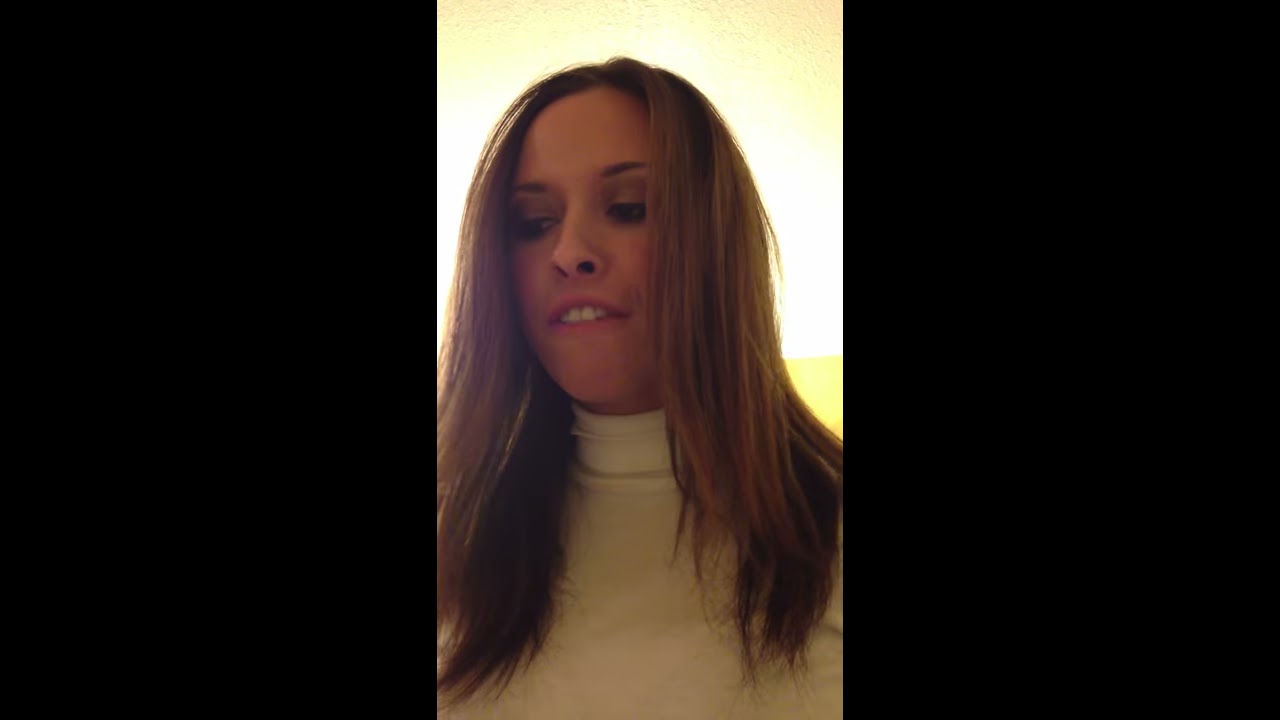The image showcases a young woman in a close-up portrait, possibly a screenshot from a video frame due to its poor quality and pixelation. This female figure, with auburn to rust-colored hair cascading just beyond her shoulders, is wearing a very snug white turtleneck. Her hair appears layered, with shorter sections at the front, possibly remnants of bangs. She wears a faint pink lipstick and gazes off to her right side imperiously, her nostrils slightly flaring and her upper teeth visible above her lower lip, suggesting she might be about to speak. The background is a nondescript, well-lit white wall, with some faint hints of yellow. The lighting on top of her head and behind her creates a strong highlight, contributing to the blown-out appearance of the image.